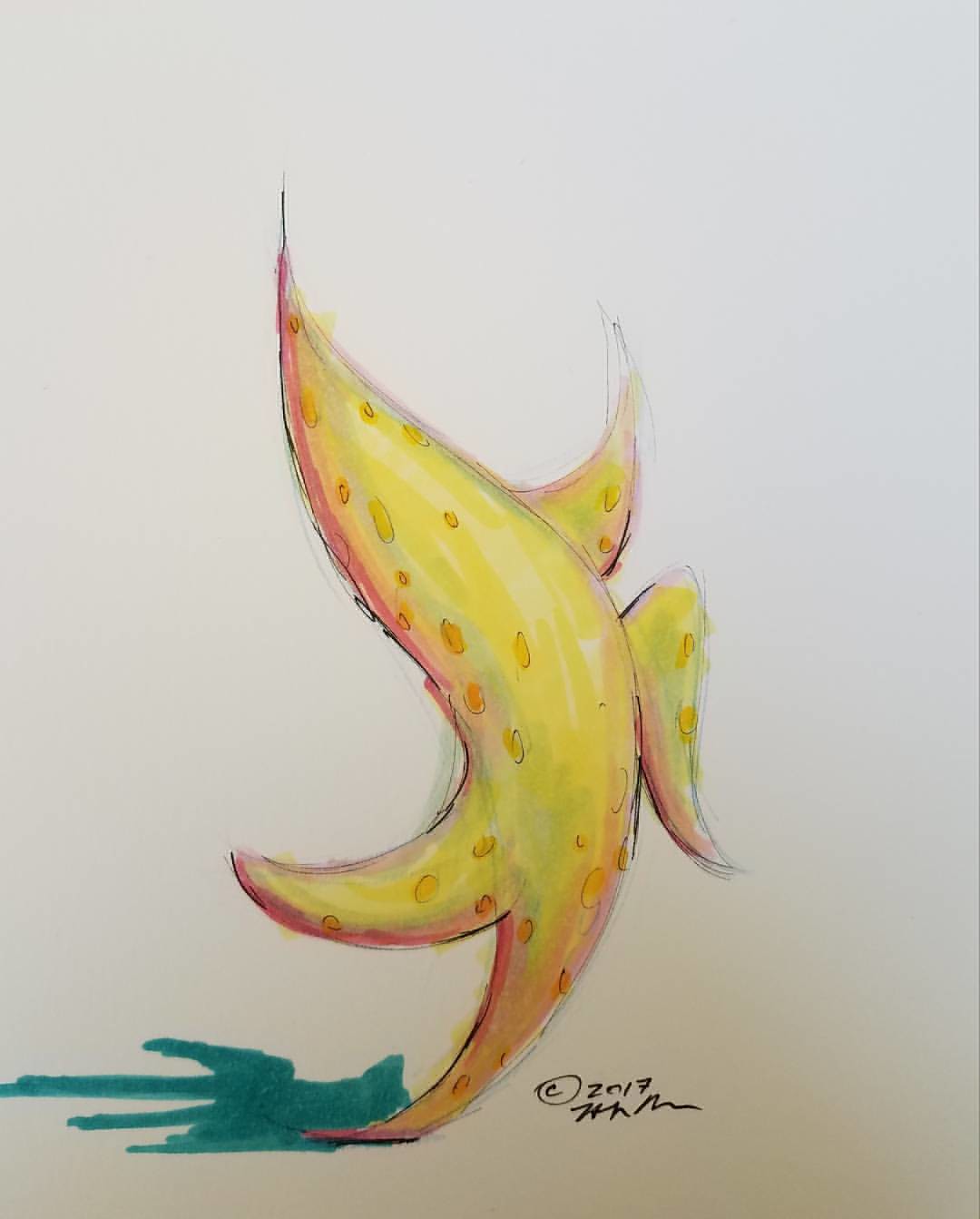The artwork, a colored pencil drawing enhanced with watercolors, is set against a cream background. It presents an abstract yet intriguing image resembling a bright yellow starfish, but with the playful charm of a skipping banana. The starfish-like figure, radiantly yellow, has five points: one point grounded, another bent upwards as if in motion, two extended to the sides, and the final point elevated as though it represents a head. A subtle green shadow complements the figure, creating depth and a sense of movement. This captivating piece, copyrighted in 2017, is signed with the initials H.N.M.